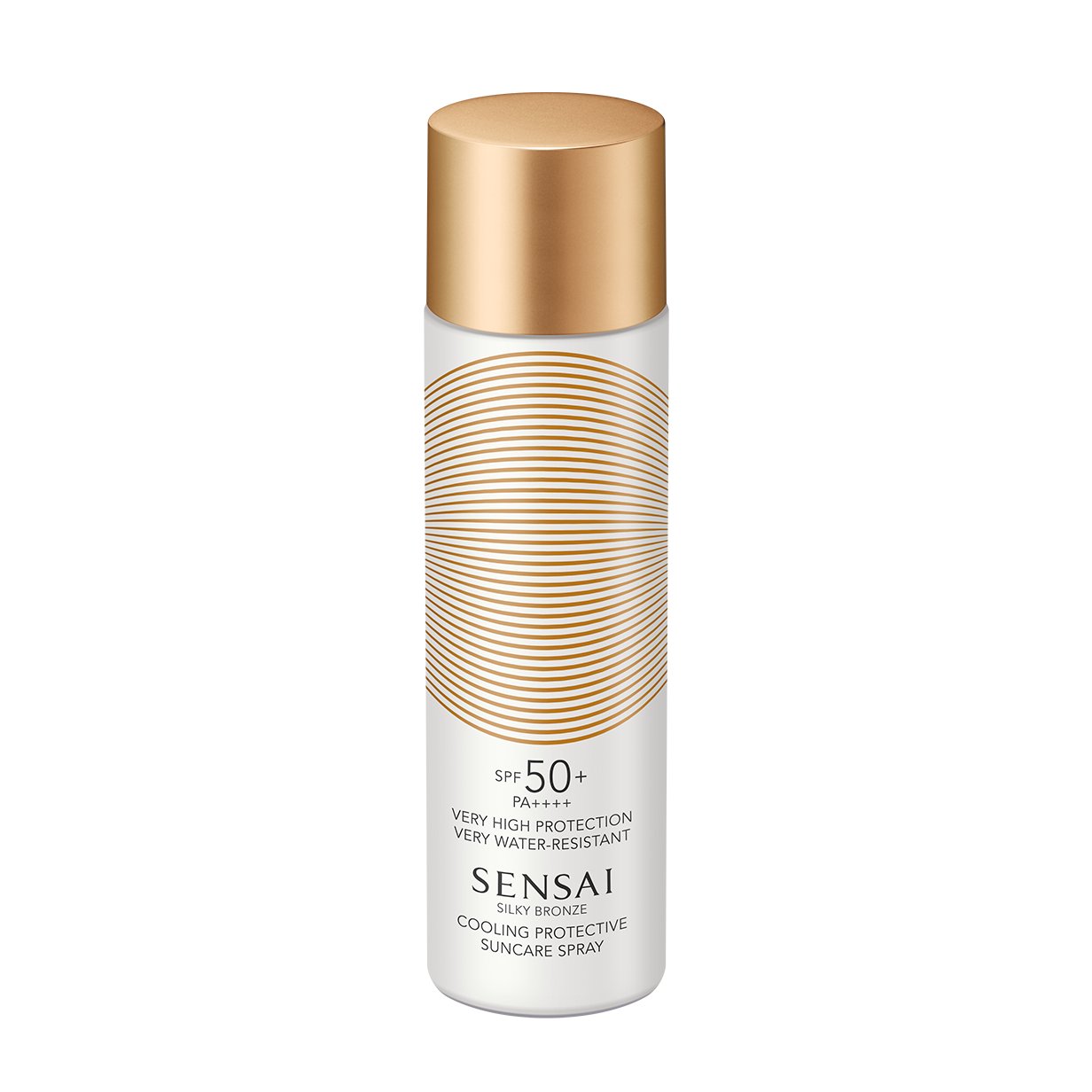The image features a tall, slim, white can with a bronze-gold cap. The cap is simple and plain in design. The upper portion of the can showcases a circular design made up of multiple, fine, gold stripes. Below this decorative element, important product information is displayed in black and gray, high-end, capital block-type lettering: "SPF 50+, PA++++, Very High Protection, Very Water Resistant." The product is named "Sensai Silky Bronze Cooling Protective Sun Care Spray," and the entire label design exudes a sense of premium quality. The can sits against a pristine white background, emphasizing its elegant and sophisticated appearance.